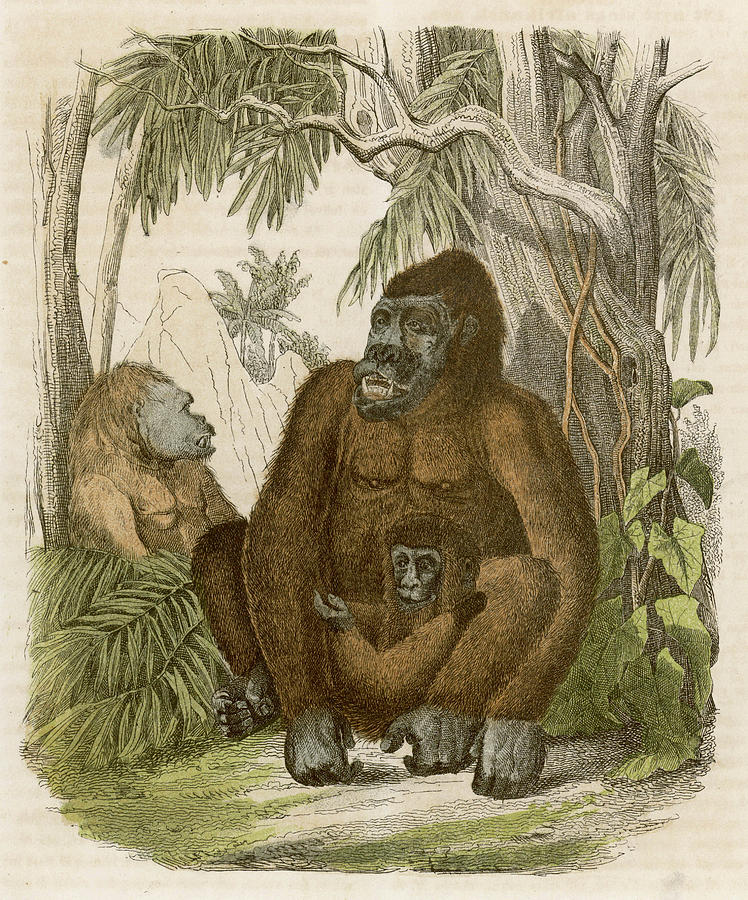This hand-drawn illustration, reminiscent of something you might find in an old 1800s or early 1900s textbook, depicts a detailed scene featuring gorillas. The yellowed paper of the illustration suggests it is quite aged. Central to the image is a large, brown-furred gorilla with darker, almost black, face, hands, and feet. This gorilla has noticeable large fangs protruding from the bottom of its mouth and is seated with a small baby gorilla nestled between its legs, mirroring the adult’s dark grayish-black colorations. Both are gazing to the left. To the left of this pair, leaning against a tree with bark of dark gray, beige, and tan hues, is another gorilla with lighter, beige or light brown fur. This gorilla shares similar facial features but only the upper part of its body down to just below the chest is visible, partially obscured by leaves. The background is completed with additional grayish trees and tropical foliage, setting a naturalistic and serene environment for these creatures.